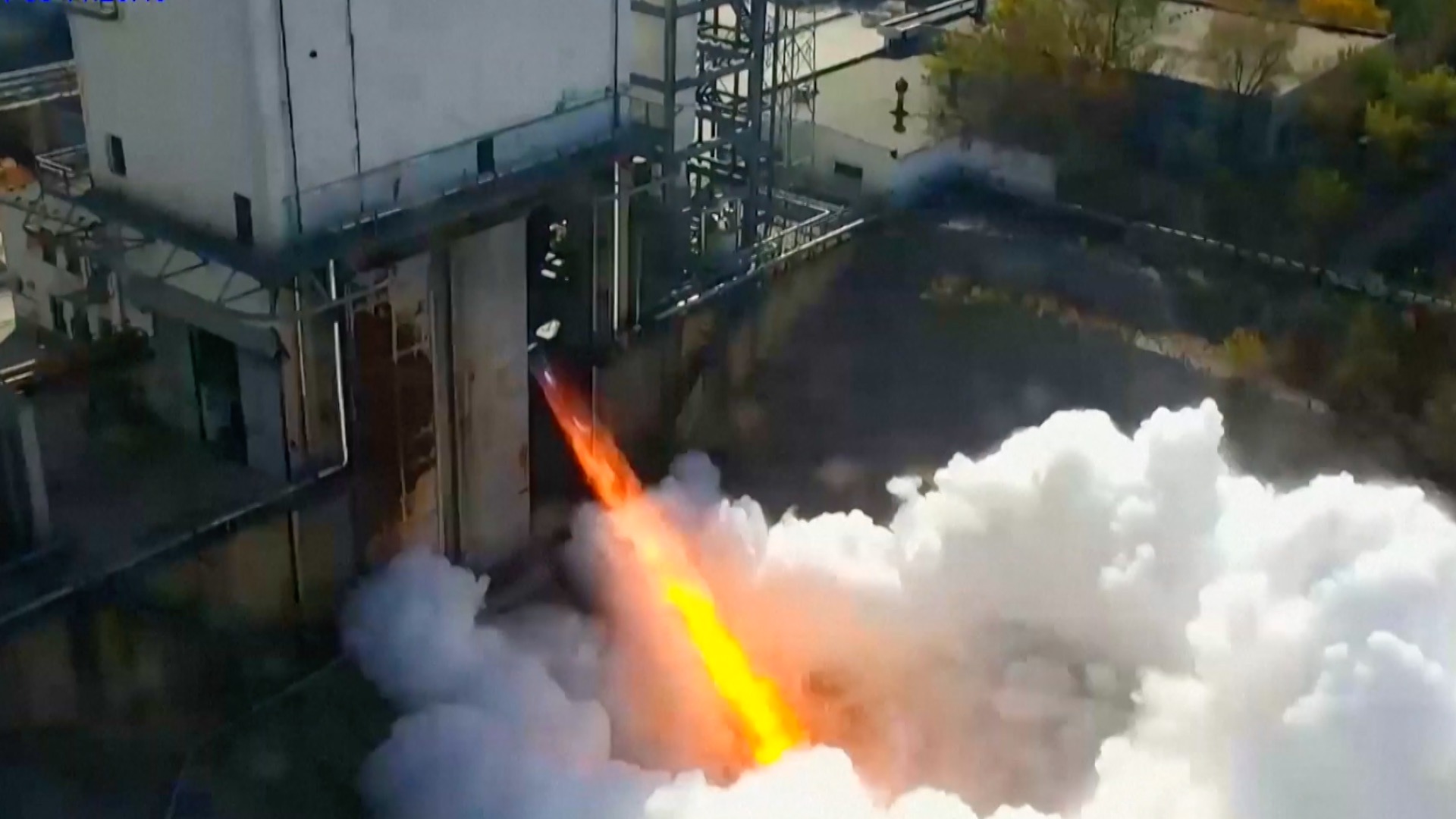This aerial photograph captures a test structure, likely for engines, positioned prominently on the left side with a large concrete and metal tower. A distinctive feature of this structure is a rectangular doorway at its base from which a powerful, streamlined flame emanates, transitioning from a bright orange at the top to a vibrant yellow further down. The flame appears to generate a significant amount of white, billowing smoke—massive, puffy clouds that resemble those seen in the sky—concentrated in the lower right section of the image. The camera's perspective emphasizes the orderly arrangement of metal ladders allowing access to different levels of the structure, surrounded by typical industrial architecture and scattered green shrubbery further right, outside the immediate area. The result is an impressive scene of industrial activity, centered around the visually striking flame and its accompanying smoke.